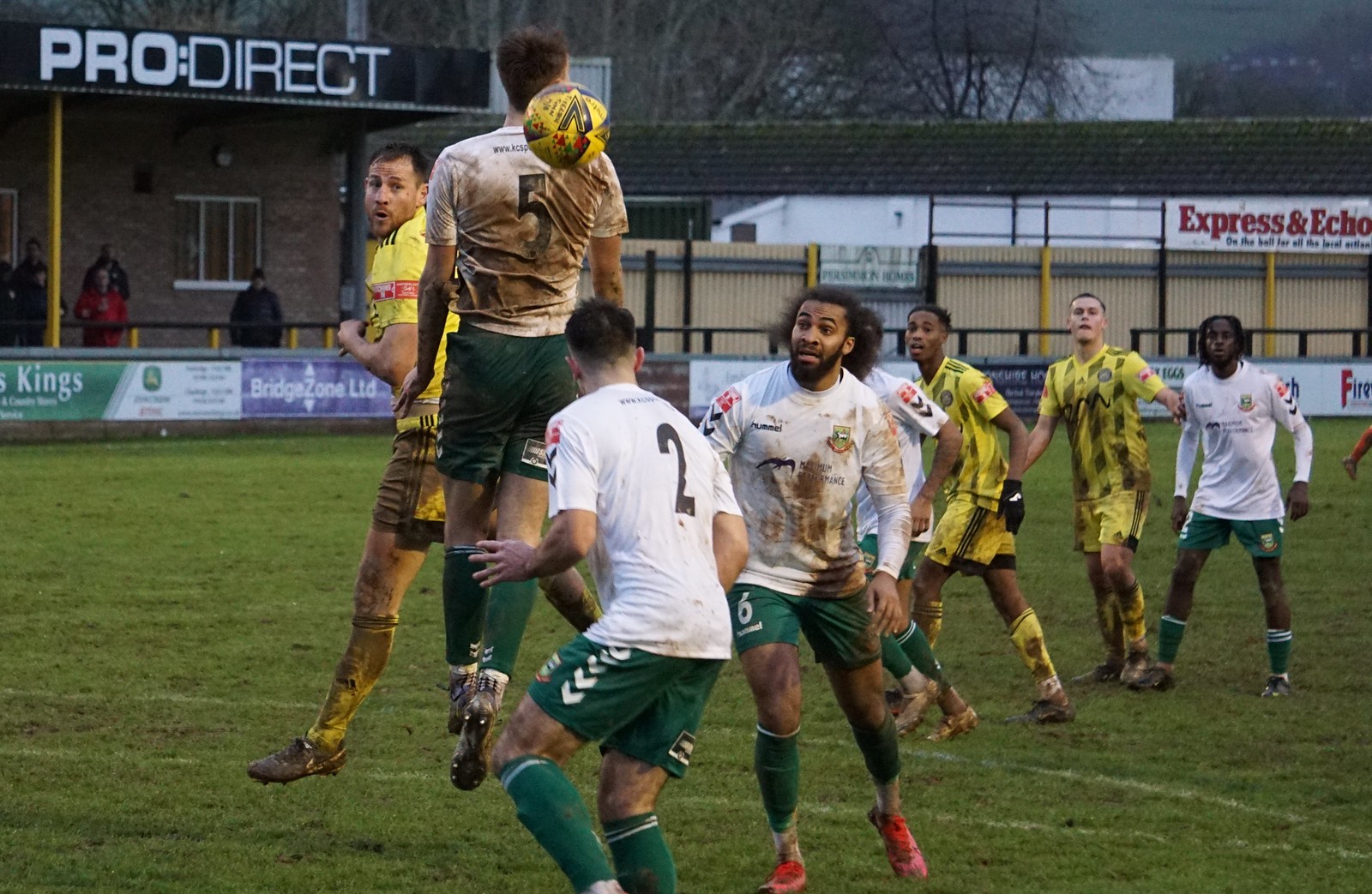This full-color photograph vividly captures a dynamic rugby match in progress. The scene features eight men, visibly muddy from their intense play, competing on a green field under a dark, grey sky. The players are split into two teams: one team sports white shirts and green shorts, while the other wears yellow shirts with black vertical lines paired with yellow shorts. 

Central to the image, a player in a yellow uniform leaps into the air, with the rugby ball positioned just behind his neck. All eyes are on him, highlighting the momentous action unfolding. Everyone on the field appears to be in motion, adding to the dynamic energy of the scene. 

In the background, a white building with a brown roof can be seen, adorned with banners. Notable signage includes "Pro Direct" and "Express and Echo," anchoring the game in a professionally sponsored setting. Despite the darkened sky, which adds an almost dramatic tension to the image, the scene is likely captured during the day, showcasing a quintessential moment in rugby.